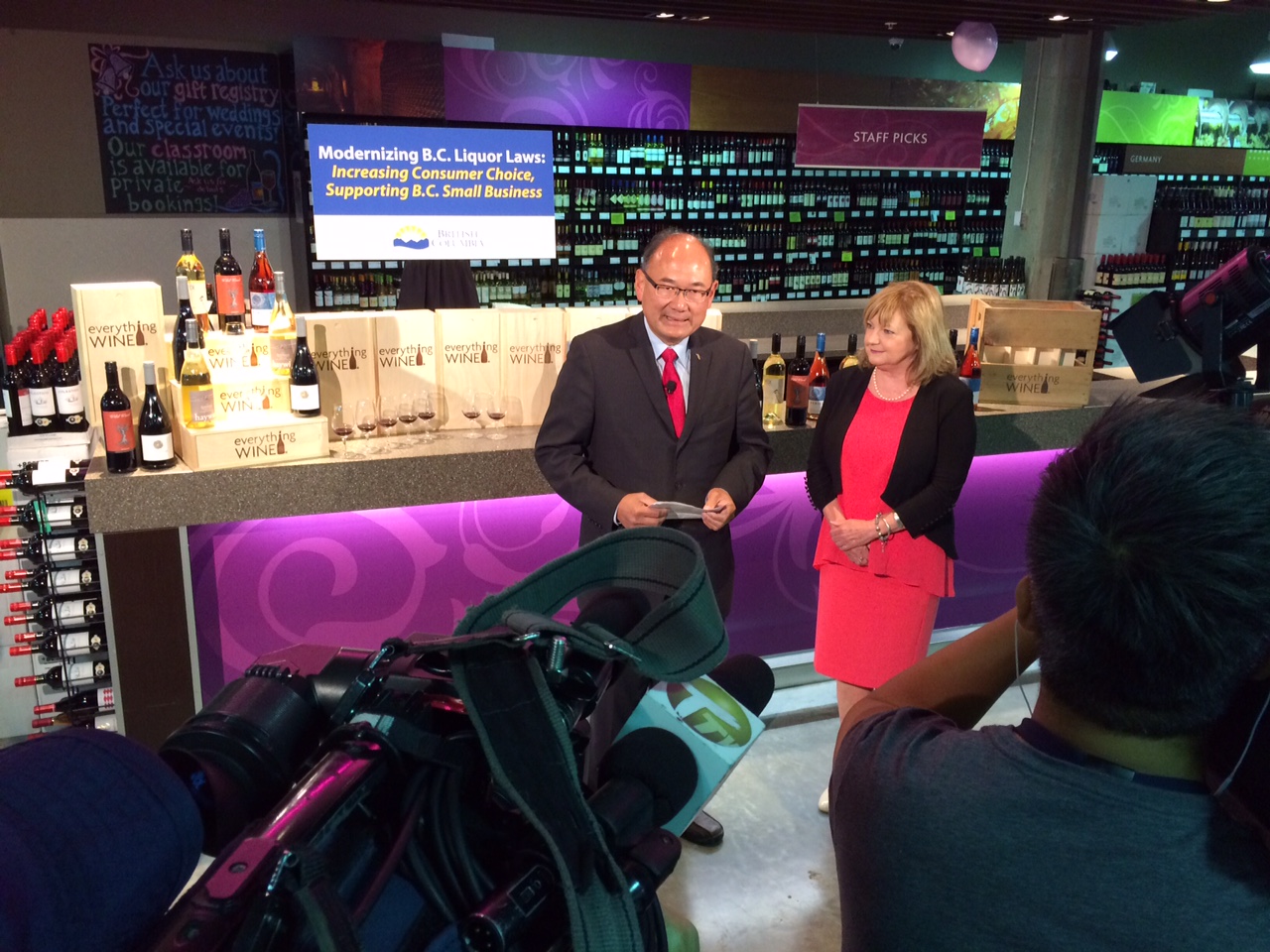The image captures a scene set on what appears to be a local news program or television show. In the foreground, professional cameramen maneuver their cameras towards two individuals standing prominently on a floor. On the left is an elderly man clad in a brown suit, a blue business shirt, and a red tie. He holds an informational card in his hand. Beside him, to the right, stands a woman dressed in a pink dress and a black cardigan. Behind them is a large counter adorned with various boxes and bottles of wine meticulously arranged in a display, including a pyramid-shaped arrangement of eight wine bottles beside the man, with a box labeled "Everything Wine" positioned among them. Additionally, a big-screen TV prominently displays the text: "Modernizing BC liquor laws, increasing consumer choice, supporting BC small businesses."